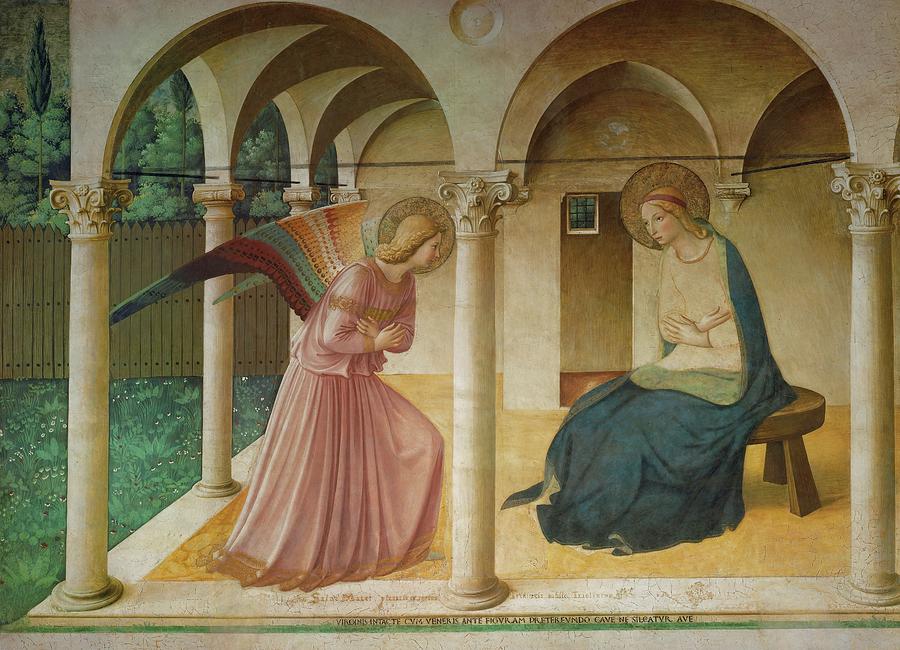This image appears to be a meticulously detailed Renaissance-style oil painting often seen as a mural in a church. Set in an outdoor patio with a tan stone roof and arches supported by columns, the scene is imbued with spiritual and artistic significance, likely representing a biblical event. 

Under the overhang sits a woman, possibly the Virgin Mary, on a wooden stool. She is dressed in a blue gown with a yellow top and has her arms crossed over her chest, directing her gaze to the left. A subtle halo hovers over her head, enhancing her sacred depiction. Opposite her, on the left side of the painting, is a kneeling angel adorned in a bright pink robe and with multi-colored wings in hues of orange, green, and red—a rare and striking feature. The angel also has a halo, blonde hair, and similarly crossed arms, looking up to the right at the seated woman.

The serene patio setting features a lawn of grass bordered by a fence, contributing to the peaceful atmosphere. At the bottom center of this mural, Latin inscriptions add a rich historical and cultural context to the scene.